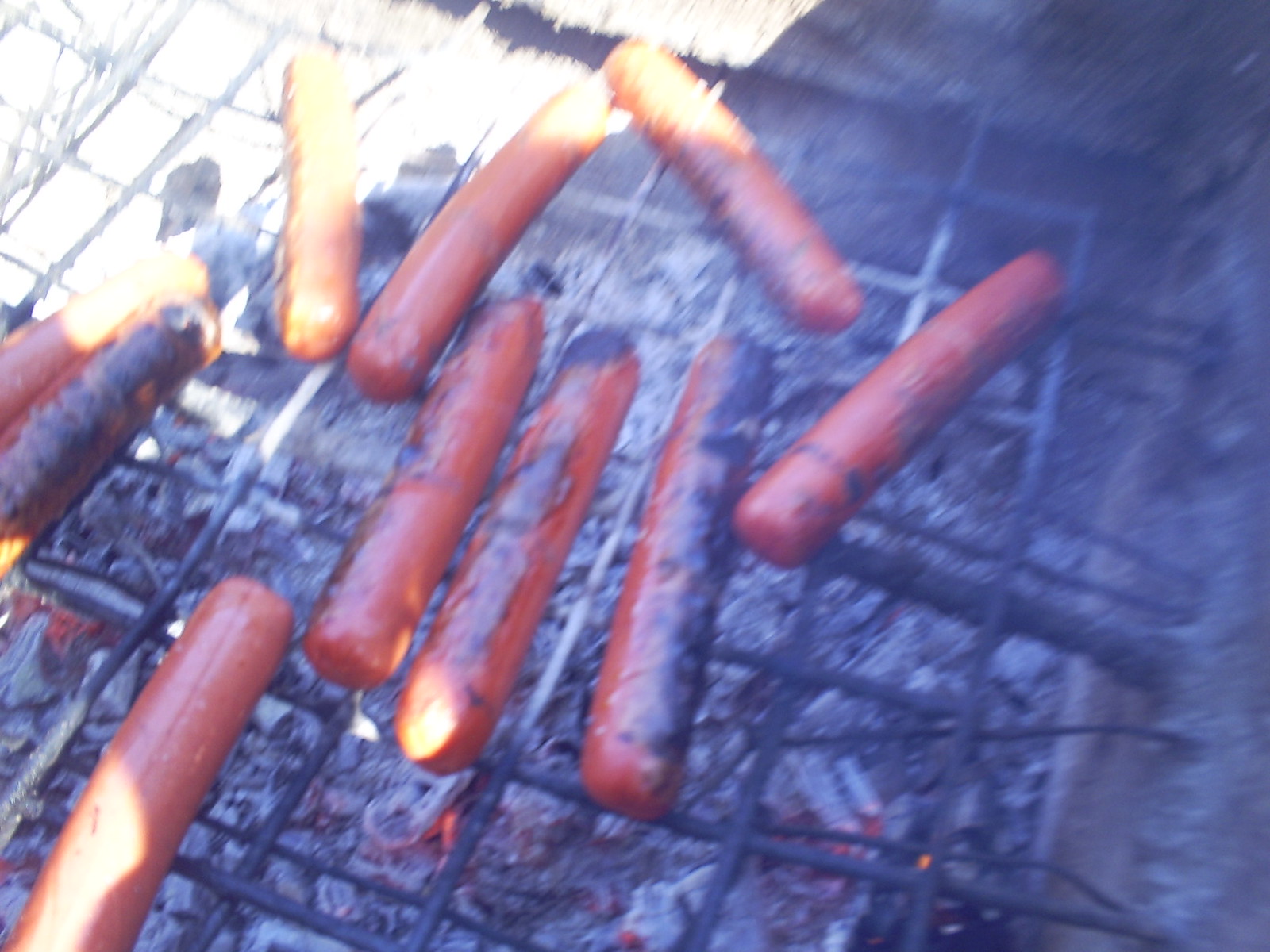This image showcases an overhead view of a large, rusted, and crusty charcoal grill, likely situated in a public park. The grill's metal bars, arranged in a slight diagonal from left to right and right to left, frame a cooking area scattered with ten hot dogs in various stages of grilling. The coals below the grill are a mix of gray ash and glowing red, indicating active cooking. Among the hot dogs, two are severely charred with blackened and bubbled up surfaces, while a few others still retain a fresh, pink hue, suggesting they were recently placed on the grill. The remaining hot dogs are a mix of pink and black, showing different levels of doneness. Both the sides of the grill and the charcoals beneath are visibly old and worn, adding a rustic feel to the scene. Amidst the scattered hot dogs, there are some placed in rows, highlighting their random yet plentiful arrangement, promising a hearty meal for someone soon.